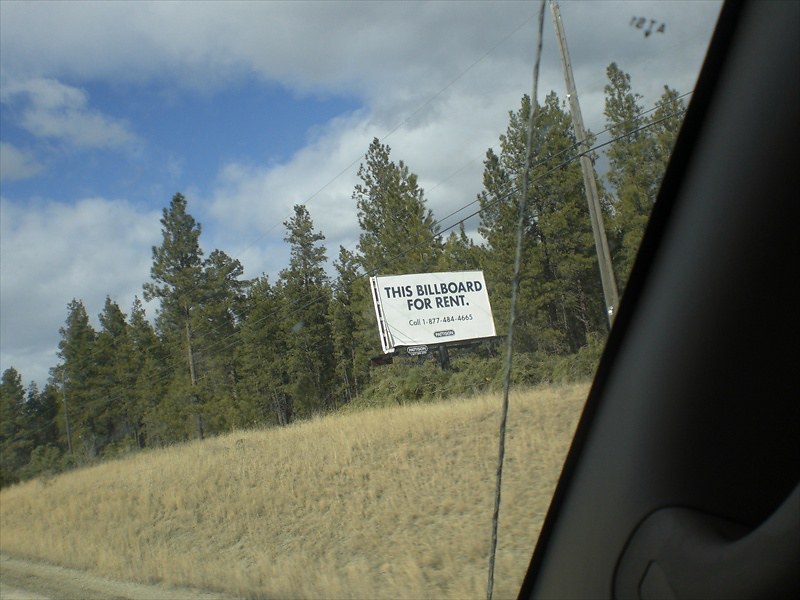A photograph captured from the passenger side of a moving vehicle, angled downward through the windshield, reveals a dynamic roadside scene. On the left, part of the vehicle's interior is visible, indicating the photo's inside perspective. The image predominantly features a stretch of highway bordered by numerous utility lines bearing several power cables. In the background, a bank with dry, brown grass clings to the side of the road. Just ahead, situated at the edge of a sparse tree line before the bank, stands a prominent white rectangular billboard. The billboard, in large black lettering, advertises "This billboard for rent," followed by a contact number underneath: "Call 1-877-484-4863 or 4663." The juxtaposition of industrial elements with natural surroundings provides a candid glimpse into roadside America.